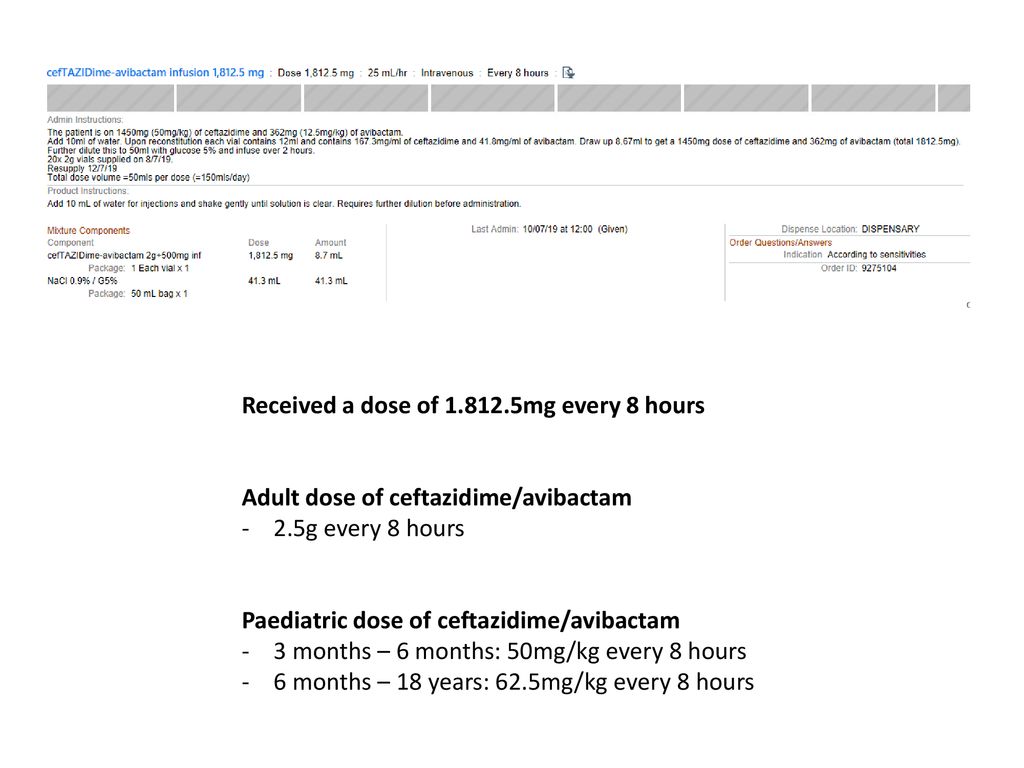The image contains medical information for dosing CefTAZidime-Avibactam. At the top, there is a series of seven gray rectangles. Above these rectangles, in blue text, the label reads "CEFTAZIDIME-AVIBACTAM infusion 1.8/1.2.5 mg dose 1.8/1.2.5 mg 25 mg/L or 20 mL per...". The text becomes blurry, but it mentions intravenous administration every 8 hours, possibly every 6 hours as well. 

Beneath this, there is more text that is too small to read clearly. Following this section, the label reiterates the dosage: "Received the dose of 1.8/1.2.5 mg every 8 hours". 

Further down, the description specifies "Adult dose of CEFtazidime-AVibactam: 2.5 grams every 8 hours", which is written in bold. Furthermore, it highlights the pediatric dose: "Pediatric dose of CEFtazidime-AVibactam for ages three months to six months."